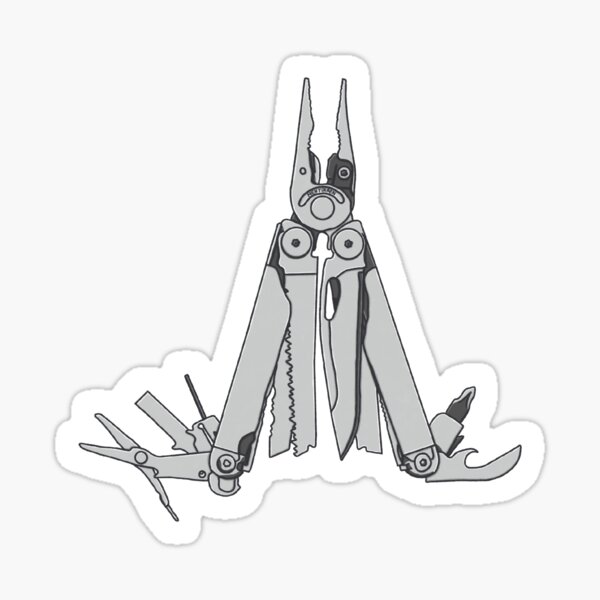This detailed black-and-white drawing depicts a multi-tool, outlined as a sticker against a light gray background. The central feature is a pair of needlepoint pliers, prominently shown in the open position. Each handle of the multi-tool contains an array of slots housing various tools. On the inside of the left handle, there are two different types of serrated blades designed for sawing. The inside of the right handle houses two sharp knife blades. Additionally, the exterior ends of the handles reveal more attachments: the right handle features a bottle opener, a Phillips screwdriver, and a thin metal poker, while the left handle contains a pair of small scissors, a file, and a screw bit. The entire image, with a vivid white cloud-like outline around the tool itself, serves as a detailed artist's rendition, emphasizing the multi-tool's versatile nature, blending practicality with intricate design elements.